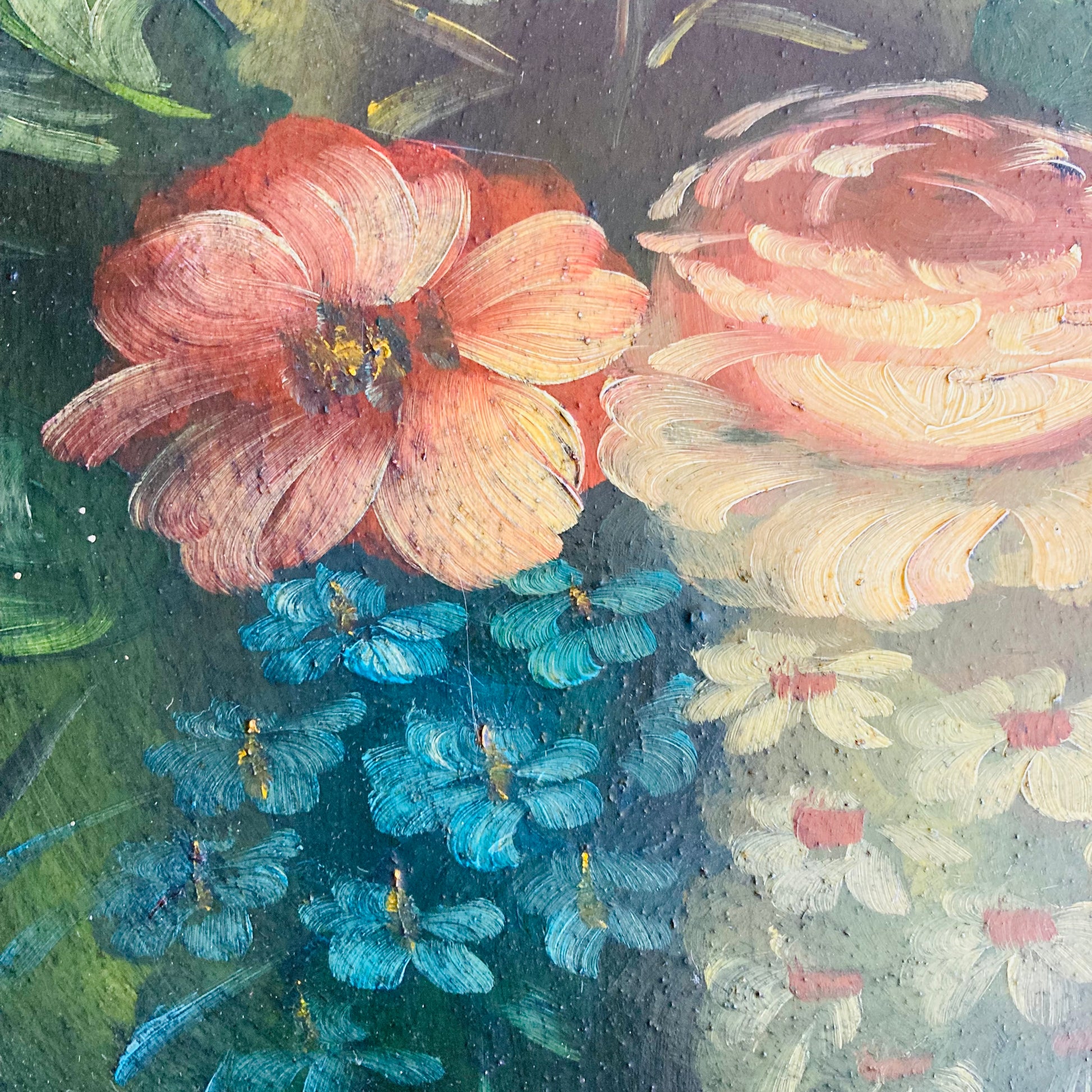The image is a detailed painting on a textured, square canvas created using dark-colored oil-based paint with visible brushstrokes. The composition features multiple, vibrantly colored flowers against a backdrop of green and brown leaf foliage. In the upper left corner, a large, striking flower with six pink petals tipped in red and a yellow filament in the center dominates, while below it, clusters of smaller blue flowers with curly yellow and brown centers add contrast. The upper right corner highlights a singular, half-bloomed rose with white petals blending into pink and red, seamlessly integrating into the green foliage backdrop. Finally, the bottom right corner displays six to seven white flowers, each with a striking red center, whereas the bottom left corner features more blue and white flowers with yellow filaments at their core. The painting's overall impressionistic style captures a free-flowing, almost floating essence of the flowers, creating a vivid and dynamic floral tableau.